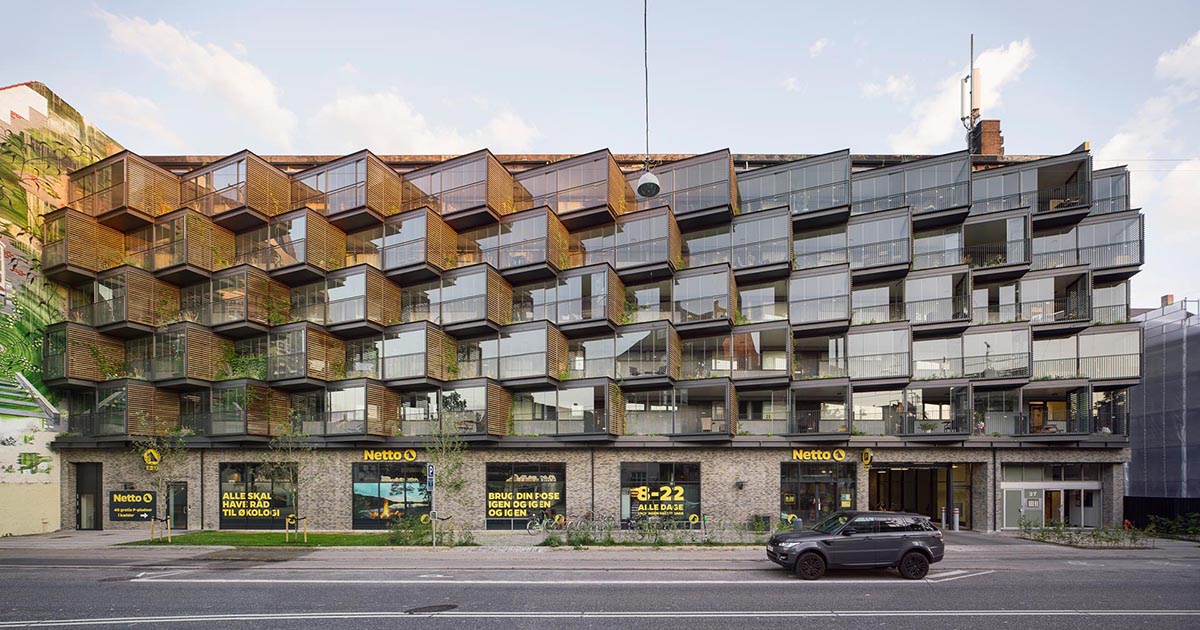The photograph captures a truly unique six-story building with a captivating blend of architectural elements. The lower level features a shop named "Netto" with its operating hours displayed in yellow on the windows. Adjacent to it on the right is the entrance to a parking garage. A dark gray SUV is parked on the street in front of the building, positioned to the right of the garage entrance. The street, with a visible road, runs in front of the structure.

The most striking aspect of the building is the upper levels, consisting of five stories of cantilevered, glass-enclosed cubicles that protrude in various directions, resembling large, transparent boxes or moving crates. These glass cubicles primarily function as apartments, each showcasing floor-to-ceiling windows, with some featuring balconies. The building is juxtaposed against another structure to the left, and the background highlights a clear, sunny day with a blue sky and scattered white clouds, along with additional constructions such as a large factory.

The left side of the image also shows a wall with some greenery, adding a touch of nature to the urban setting. Antennas on top of the building complete the scene, suggesting a mix of residential and commercial utilities within this intriguing architectural marvel.